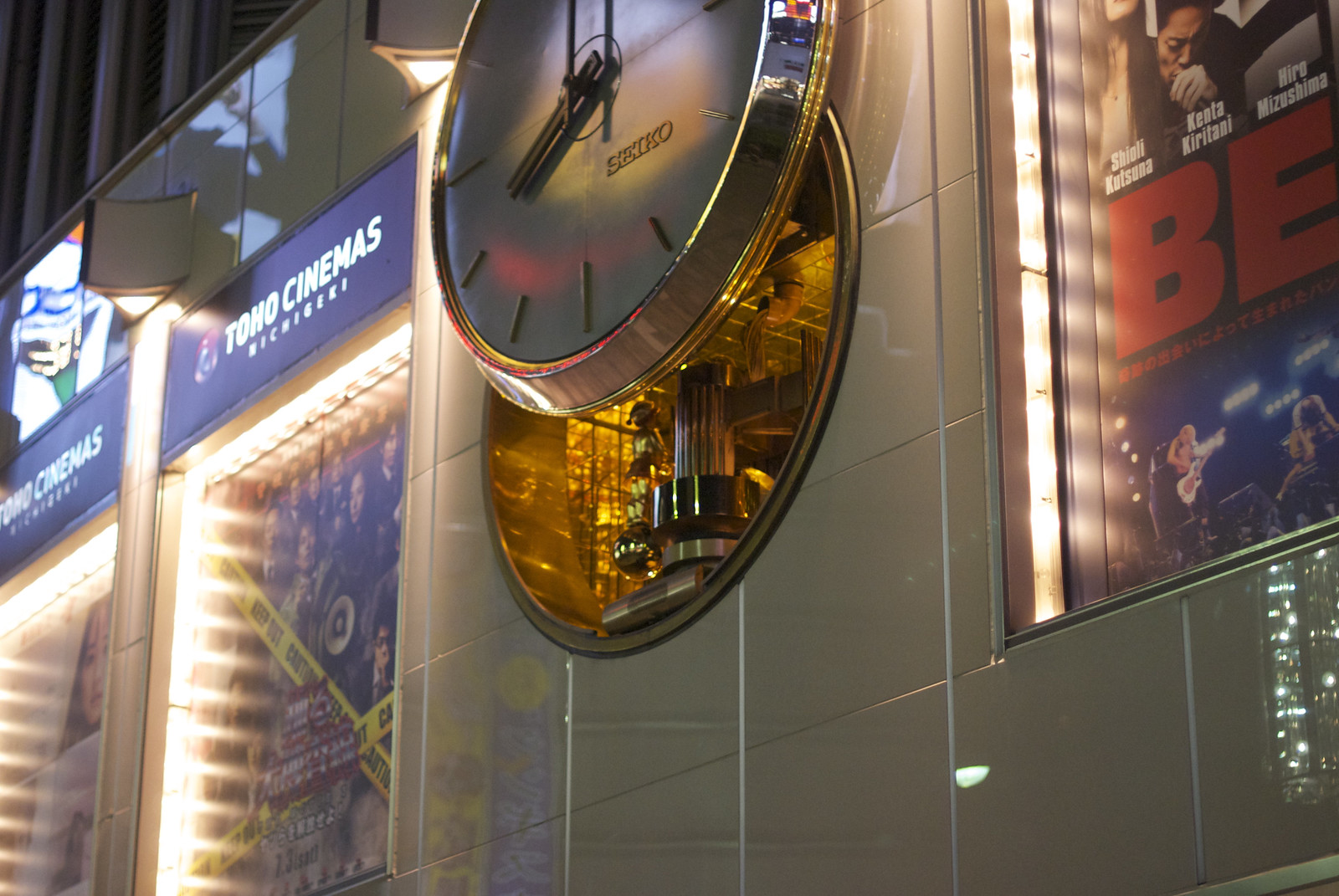The photograph captures an exterior view of a movie theater, prominently showcasing a large clock centered on the building's facade. The clock features a unique design with a slightly recessed face, providing a glimpse into its inner mechanisms. Flanking the clock are three movie posters under the label "Tono Cinemas," indicating the theater's name. To the left of the clock, two indistinguishable movie posters are visible. To the right, a third poster displays the partially visible title "B.E." in bold red capital letters, accompanied by white text listing the actors' names just above the title.